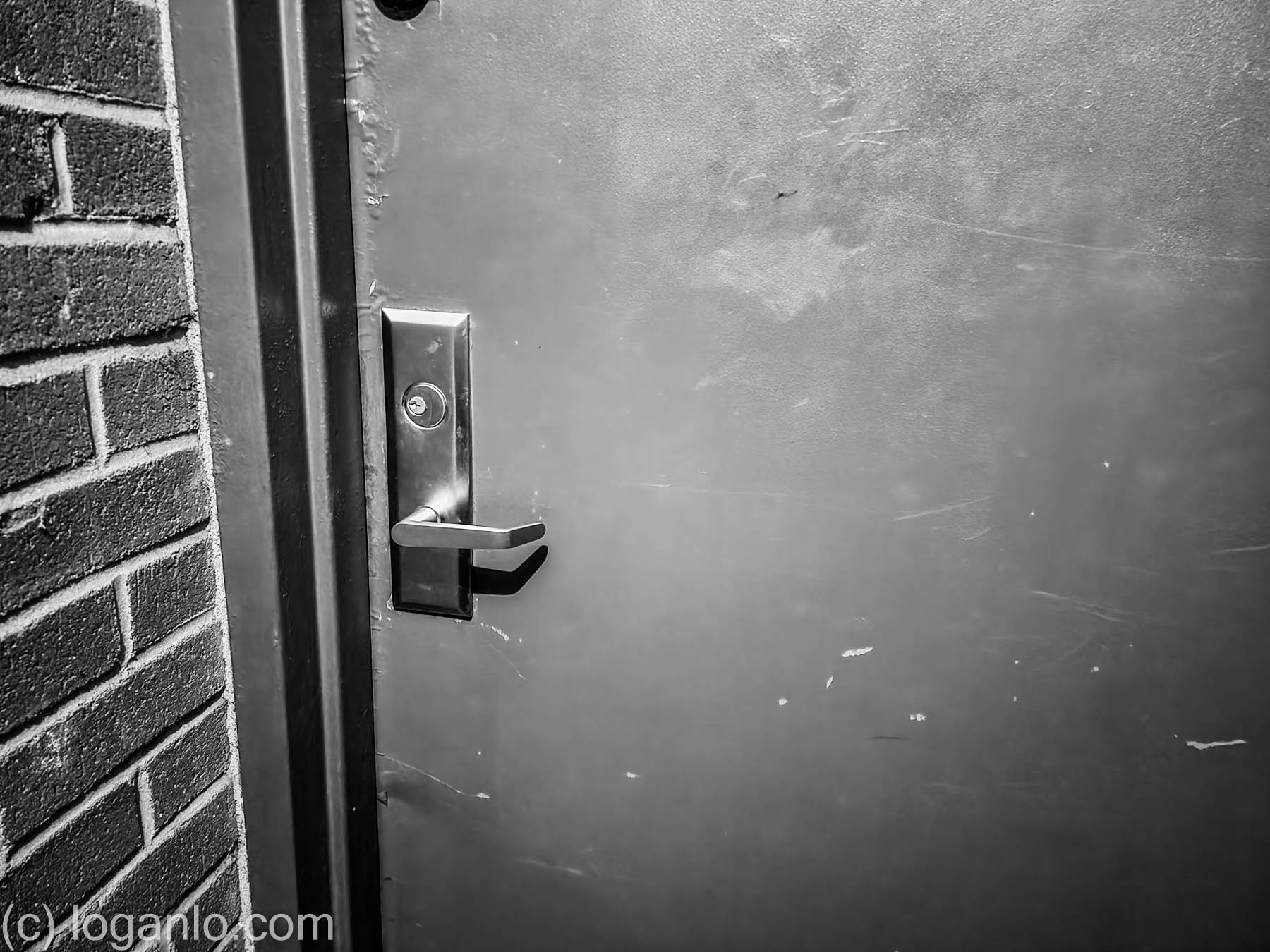This photograph presents a close-up view of a weathered, old door, conveying a rich history through its numerous imperfections. The door, painted a light gray, is marred with copious scratch marks, chipped paint, and notable scuffing particularly around the silver door handle and the lock. The left-hand side of the door showcases more intense damage, suggestive of past attempts to force entry. Additional scratches accentuate this narrative of resilience against time and possible tampering. In the lower left-hand corner of the image, the copyright mark "LoganLowe.com" subtly indicates the source of the photograph. The door stands as a testament to durability despite its worn appearance, juxtaposed against a backdrop of black and white charcoal bricks that form a sturdy wall on the far left. The rough texture and evident wear of this heavy-duty door narrate a silent story of endurance and strength.